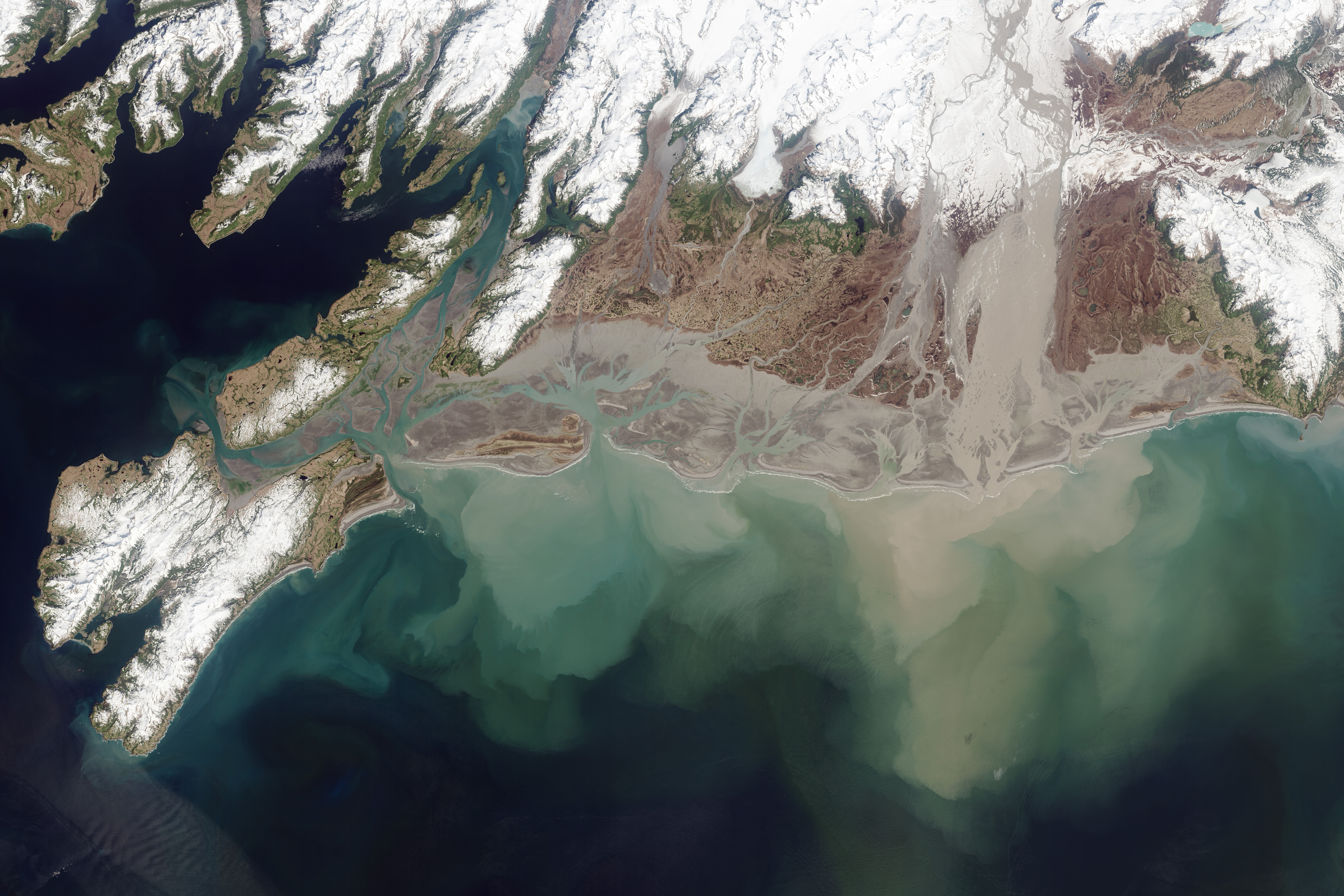This image appears to be a bird's eye view, possibly taken from outer space or at a great altitude, capturing a diverse and expansive landscape bordered by the ocean. The landmass exhibits several notable features: extensive white areas likely indicating snow-capped mountains, sprawling patches of greenery, and expanses of brownish-pink terrain. The coastline is intricately shaped, with curving edges and long ridges resembling fjords, suggesting a rugged topography. The ocean exhibits a gradient of colors, transitioning from dark blue in the deeper regions to lighter hues of blue and green closer to the shore. Additionally, a visible contaminant or sludge on the right side appears to be polluting the water, accompanied by smog-like haziness. The overall scene combines elements that might suggest both photographic and artistic qualities, adding to its detailed and complex appearance.